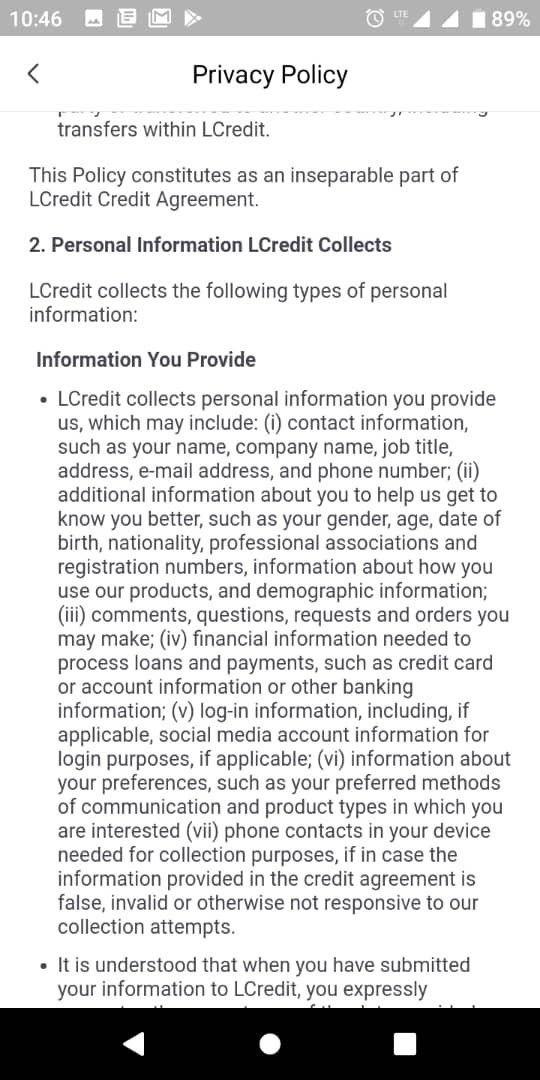This is a detailed screenshot taken from an Android phone interface. The top banner is light gray, displaying the time as 10:46 on the left. Adjacent to the time is a sequence of icons: a picture icon, followed by a paper icon with lines, and another paper icon overlapping a box. Next, there is the Google Mail icon, and an unidentified icon beside it. On the right-hand side of the banner, icons indicate a clock, LTE network status, two full signal bars, and a battery icon showing 89% charge.

Below the banner, on the left, there is a left-pointing arrow. Centrally aligned is the text "Privacy Policy". Further down, the text reads "Transfers within L Credit," which is part of a paragraph that appears to be cut off. Following this, the text states: "This policy constitutes an inseparable part of L Credit's credit agreement."

The next section, labeled as number two and bolded, reads: "Personal Information L Credit Collects." It begins with "In the beginning..." and continues to outline the types of personal information collected by L Credit. The text explains: "This is information you provide," followed by two bulleted points. The first bullet point is quite lengthy while the second one starts with "It is understood that when you have submitted your information to L Credit you expressly..." but the rest of this bullet point is cut off.

Overall, the image clearly details elements of an Android device interface while providing a glimpse into the privacy policy and personal information collection practices of L Credit.